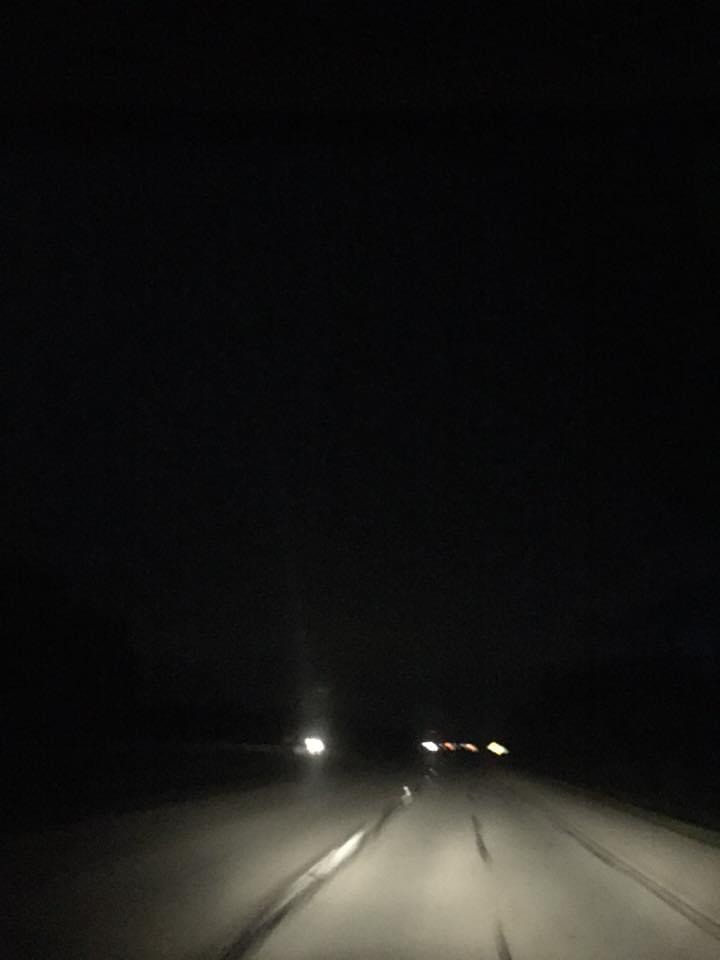This nighttime photograph captures a dimly lit, four-lane road curving slightly ahead, framed by the consistent blackness of the surroundings. The top three-quarters of the rectangular image is engulfed in darkness, emphasizing the black night sky. The bottom portion reveals a blurry but discernible road, illuminated by headlights, with a dotted gray center line marking the lanes. Ahead in the distance, there are five faint light dots, possibly from other vehicles. On the left side, a prominent white light stands out, likely from a stationary source rather than a car. The image is primarily dark with subtle shapes resembling trees on either side, enhancing the eerie and obscure ambiance. Despite the blurriness, dim medium-sized lights from what seems to be a freeway overpass are faintly visible, aligning horizontally across the scene.